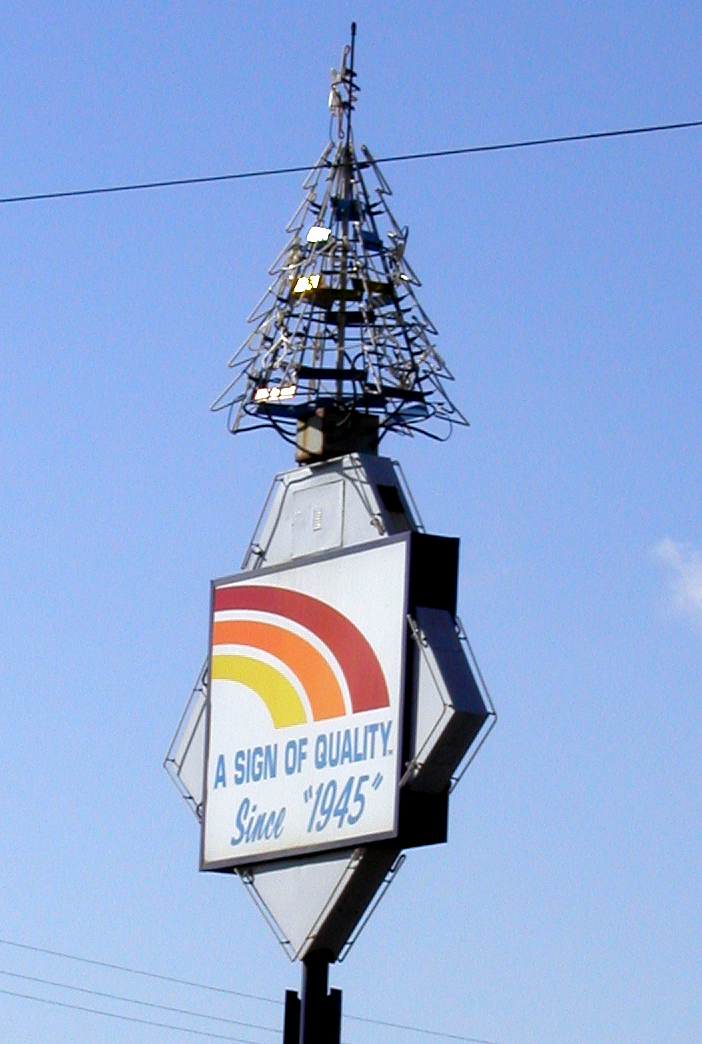This outdoor image captures a striking business sign set against a clear blue sky, with only a single wispy white cloud adding texture to the scene. The viewer's perspective is from below, looking up at the sign. At the top of the image, a power line crosses the view, and additional power lines are visible at the bottom.

The sign itself is diamond-shaped with a predominantly white background. In the center, a square contains the text "A sign of quality since 1945" in bold blue lettering. Below the text, three curved lines in yellow, orange, and red create a rainbow-like arc, adding a splash of vibrant color to the design.

At the top of the sign, there is a formation that resembles the shape of a Christmas tree, made from what appear to be neon rods. Though unlit in the daytime, these neon elements hint at a different, possibly illuminated look after dark. Additional potential neon shapes adorn the very top of the sign, completing its vintage and eye-catching appearance.